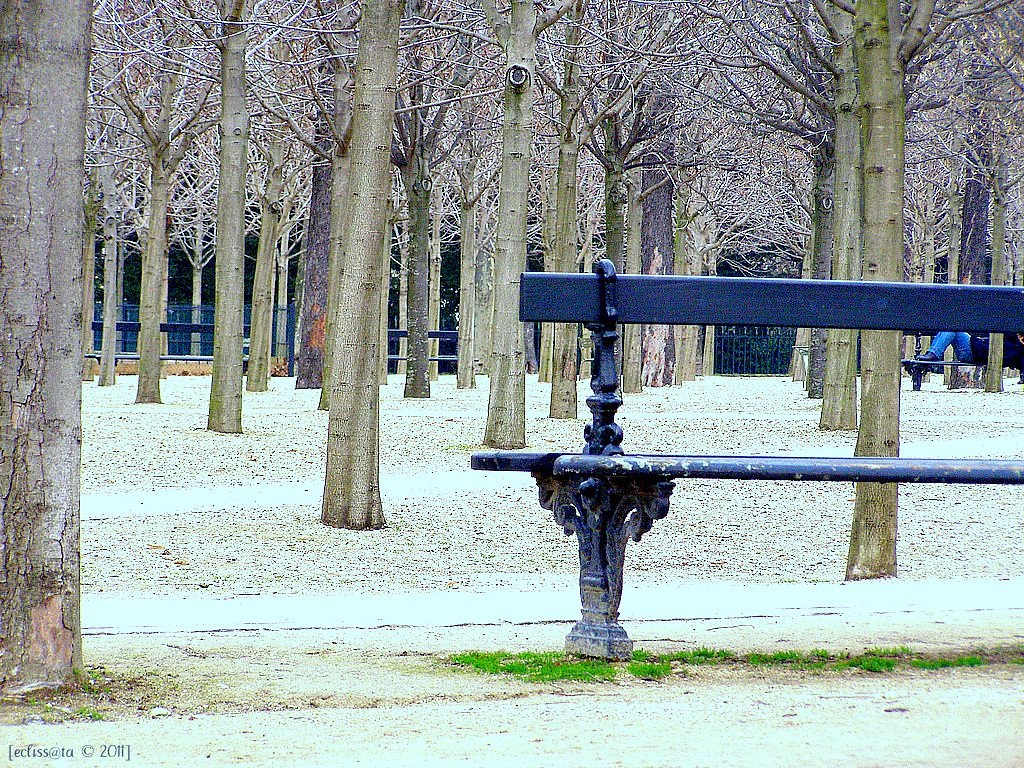The image showcases a tranquil winter park scene blanketed in a light dusting of snow, suggesting it's mid-winter or late fall. The focal point is an antique-looking blue wooden park bench with a single backboard and two planks for the seat. In front of it, you can just make out another wooden bench where someone appears to be lying down, wearing blue jeans and black shoes. This contrasts beautifully with the stark, leafless trees in the background, which seem to be perfectly aligned like in a well-maintained pecan orchard. Snow lightly covers the ground, the trees' branches and even a nearby sidewalk, while small patches of green grass peek out from under the bench. The image has a certain brightness, possibly enhanced by editing or a filter, adding to its crisp and serene atmosphere. This beautiful photograph, taken around 2011 by an artist named Ecliss, captures the pristine chill of a winter's day in the park.